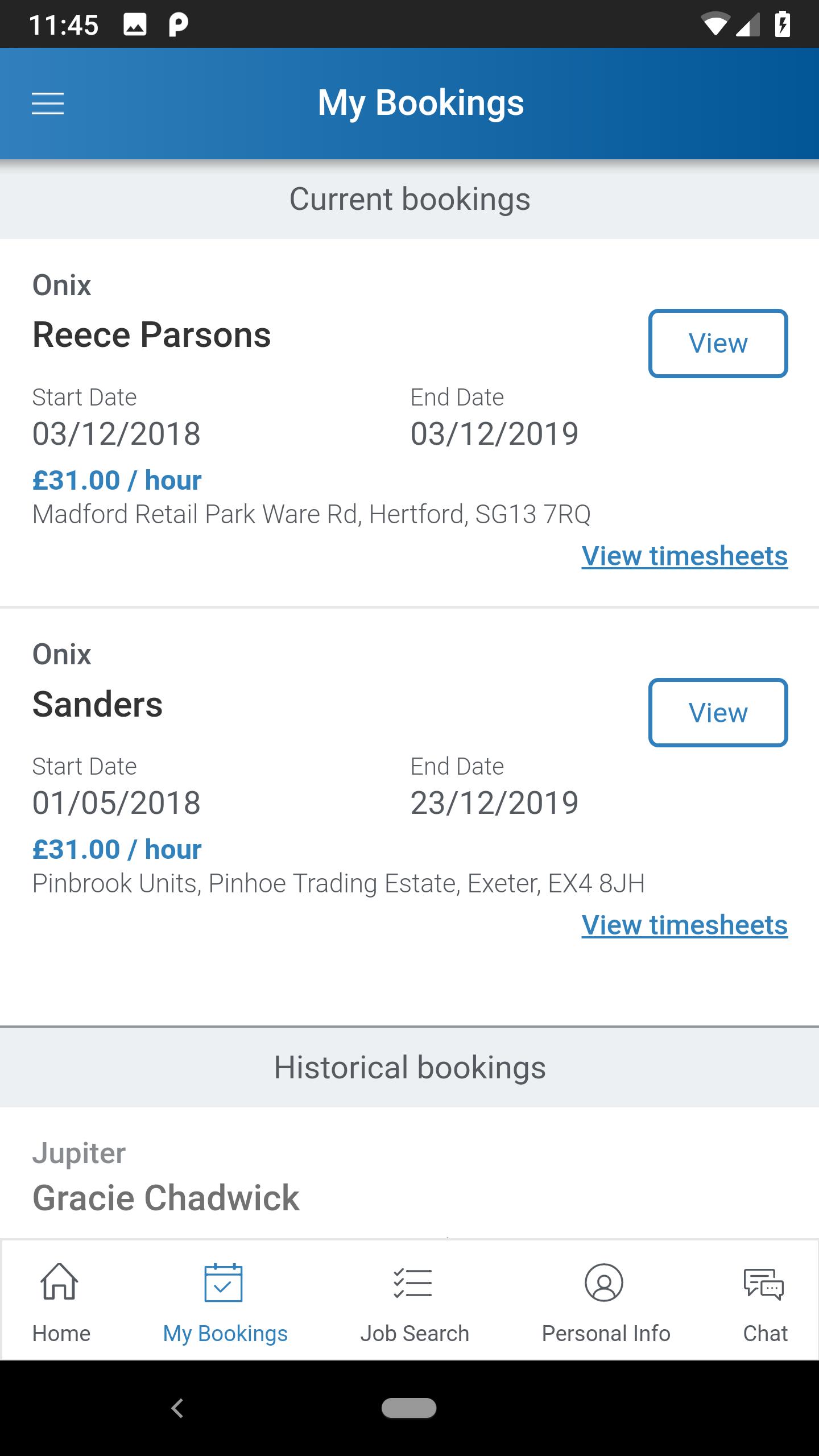This mobile screenshot depicts the user interface of a bookings app for a freelance job company, showcasing the 'My Bookings' section. The top of the screen features a dark blue header stating 'My Bookings' centered prominently. Just below the header lies a thin grey bar with 'Current Bookings' inscribed in grey letters. 

Directly underneath, a vertical list presents the user's current bookings. The first booking entry provides comprehensive information including the company name, client name, start date, end date, hourly rate, and address. On the upper right of this entry, a 'View' button is available, while the bottom right offers a 'View Timesheets' option in a blue hyperlink font.

At the screen's bottom, a grey bar labeled 'Historical Bookings' is visible, partially displaying two names from this category. The top historical booking entry shows 'Jupiter' as the company name and includes information regarding the reporting manager or the associated job.

Frequently used navigation options are positioned at the bottom of the phone's display in a panel with icons labeled: Home, My Bookings, Job Search, Personal Info, and Chat. The 'My Bookings' icon is highlighted in blue, indicating the current active section.